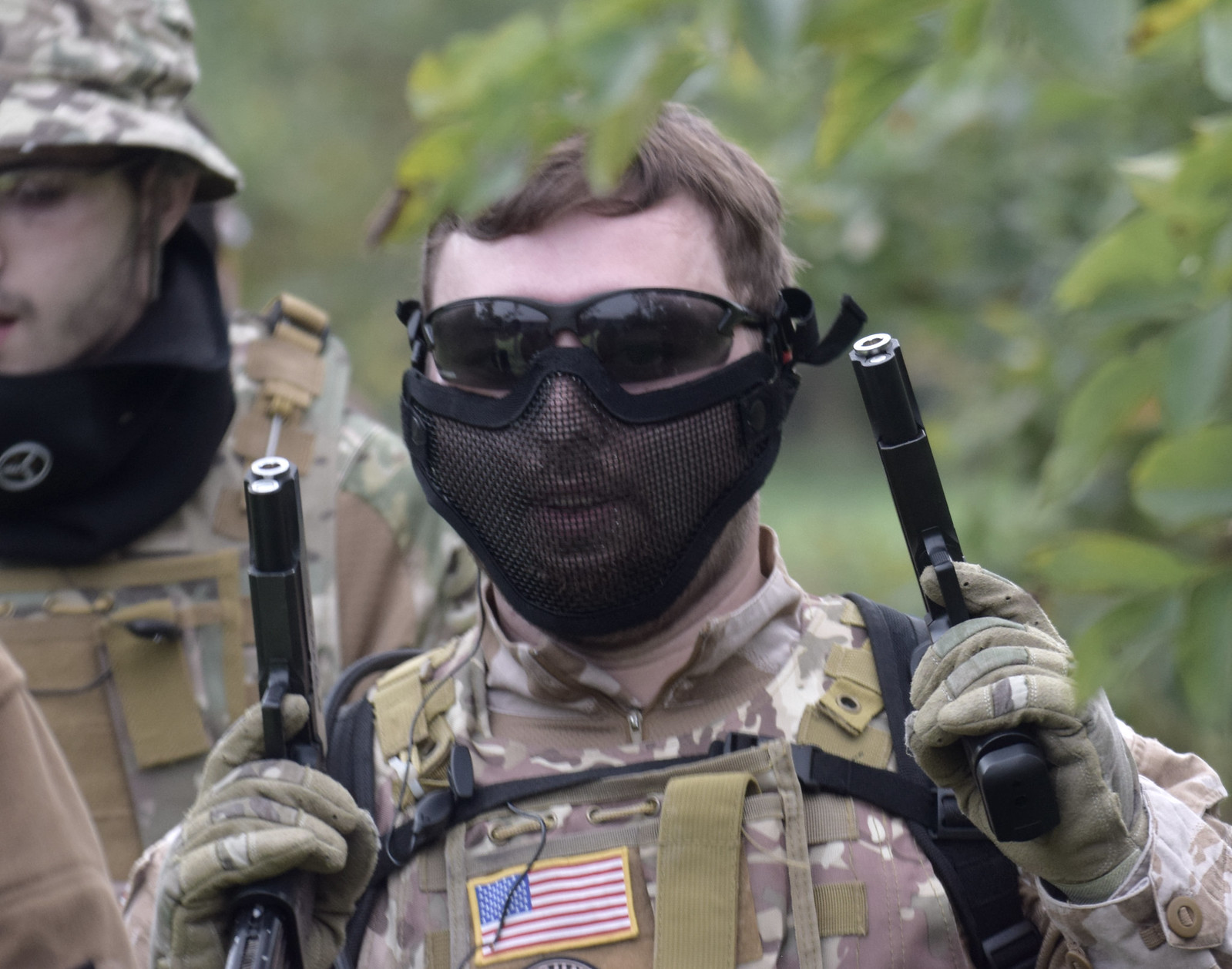In the image, two men are standing in a forest, surrounded by blurry foliage. Both are wearing camouflage military fatigues and black face masks. The central figure, positioned prominently, has short brown hair, black sunglasses, and a black mesh mask. He holds a pistol in each hand, with his fingers on the triggers. His uniform is adorned with a gold-outlined American flag patch, and he wears gloves. The man in the background is partially obscured, wearing a camouflage hat and a black scarf with a Mercedes logo. He also has a flak jacket. Although they wear military-style gear, the lack of proper insignia and non-standard grooming suggests they are not actual military personnel.